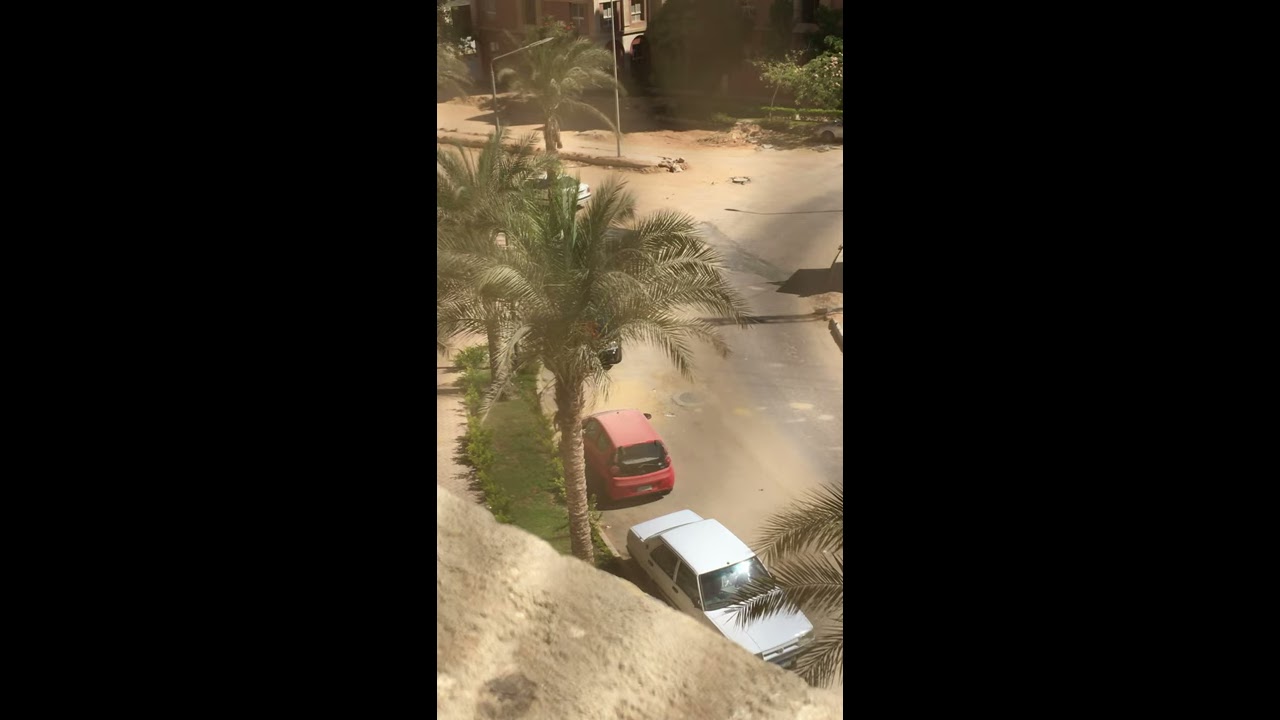This image features a central vertical rectangle flanked by solid black on either side, creating a striking contrast that draws attention to the core scene. The photograph appears to be taken from an elevated perspective, possibly from atop a sandy cliff or a balcony. It captures a desert-like environment with a sandy-brown landscape and scattered green palm trees. At the base of the image, a dusty, sandy road runs horizontally, on which two cars are parked—a medium-sized white sedan directly below the observer and a smaller, red hatchback further down the road, parked with its bumper behind the white car’s bumper. Prominent in the upper portion of the image is a street light mounted on a tall metal pole, adding to the sense of an arid, possibly remote location. The road is flanked by sporadic bushes and palm trees, adding to the desolate, sandy ambiance.